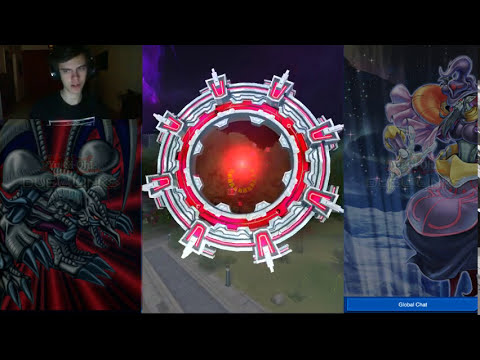The image is a screenshot from a video game, divided into three distinct sections, each framed by long horizontal black bars at the top and bottom. In the top left, there's an image of a gamer with black hair, wearing headphones, and slightly tilting his head to the left. Below him is a design or illustration of a creature resembling a metal dragon or bionic monster, featuring gray tentacles and red lines, set against a red background. The middle section showcases a striking circular disc with multiple layers: a bright orange sphere at the center with an orange background, surrounded by a gray ring, a red section, and another gray outer ring. This circular object is positioned over a landscape featuring a small sidewalk next to a green grassy field, hinting at the gameplay environment underneath. The right section depicts a peculiar purple clown-like or robot creature with a textured body and a purple belly, enclosed in a square. At the bottom of this section, a blue bar with blurry white text reads "Global Chat." A stream of light appears to emanate from below the creature.